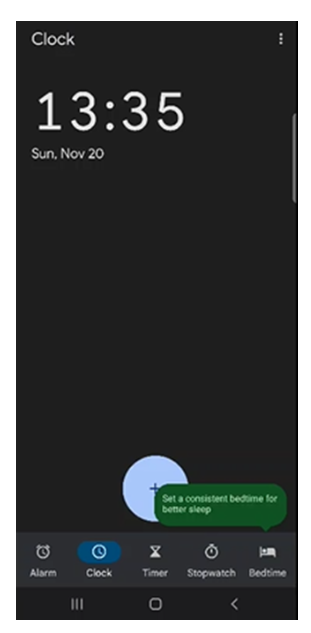A clean and detailed caption for the image described:

"The screenshot showcases a person's home screen in a primarily black theme. At the top left corner, the word 'Clock' is displayed in white text next to a three-dot menu icon. Centered on the screen is the time, formatted in military time as '13:35' (1:35 PM) in white. Directly below the time, the date 'Sunday, November 20' is shown, separating the day and month with a comma. 

At the bottom of the screen, there's a blue circular icon with a white plus sign inside, positioned just above the category options. The category options are presented as icons: an alarm clock for 'Alarm', a circular clock for 'Clock', an hourglass for 'Timer', a stopwatch for 'Stopwatch', and a bed for 'Bedtime'. Below these, there are three small circular icons arranged in a row, likely indicating additional functions or quick access tools. On the far bottom, a small home button icon and a left arrow icon are visible, serving navigation purposes."